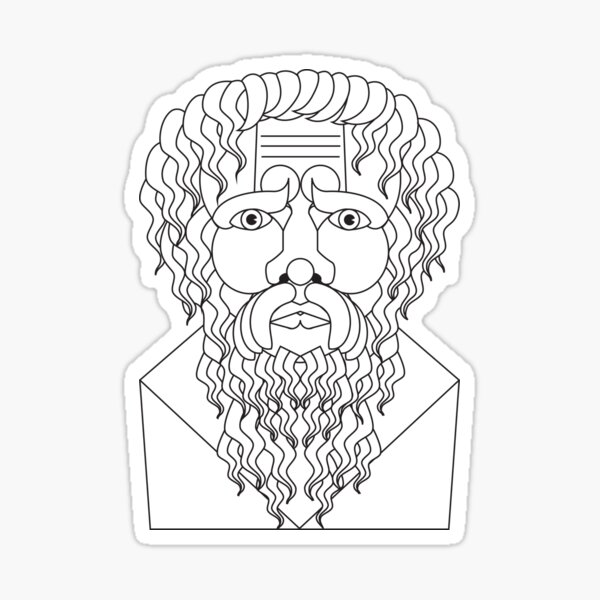This image depicts a stylized sticker of a bearded man, with a black-lined drawing on a plain white background. The figure features long, wavy hair that cascades over his forehead, which is marked by three distinctive horizontal lines. His pronounced eyebrows arch upwards, ending in circular shapes at the brow points. The man's wide-open eyes and prominent nose, which is marked by a characteristic circle, add to his serious expression. A long, flowing beard with curly, hanging strands mirrors the wavy hair on his head, contributing to a sense of intricate simplicity. The man's shoulders are broad and boxy, and he appears to be clad in a robe-like garment, evoking the classical image of a philosophical figure from the Greek or Roman era. The illustration is framed by a thin gray border, enhancing the impression of a cutout print or sticker.